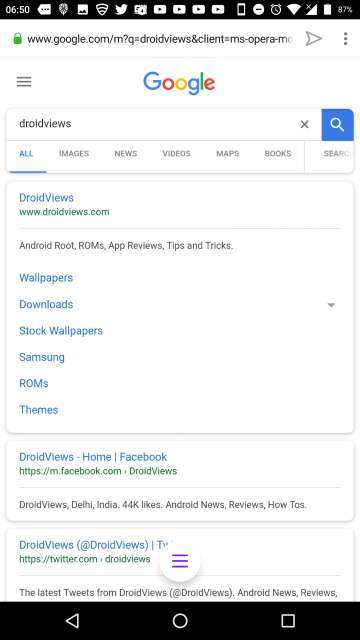The image is a screenshot taken from a cell phone displaying a Google search results page. At the top of the screen, there is a black bar with white icons, offering clear visual contrast. Centered in the black bar is the Google logo, prominently featuring its iconic colorful letters. Below this, various navigation tabs are listed: "All," "Images," "News," "Videos," "Maps," "Books," and a search area. The "All" tab is underlined, indicating it is currently selected.

Just below the navigation tabs, the text "droid views" appears in bold blue letters, indicating a search result title. Beneath this, a green URL is visible, highlighting the website's address. The URL leads to a web page dedicated to Android-related content, specifically mentioning "android root, roms, apt reviews, tips, and tricks." Within a rectangular section under this, there are six additional blue links with the following labels: "wallpapers," "downloads," "stock wallpapers," "Samsung," "roms," and "themes," suggesting further resources or sections available on the website.